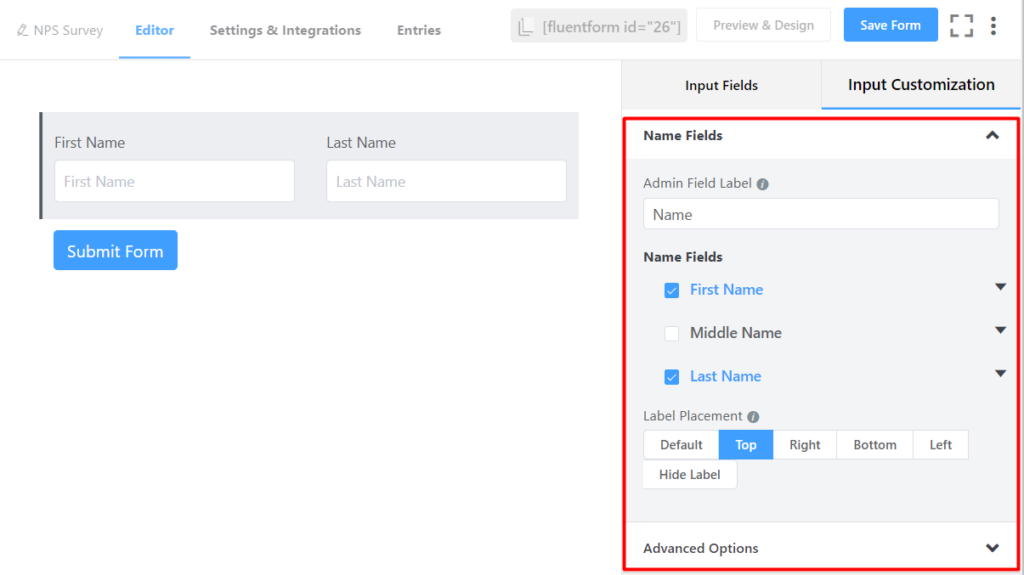To the right side of the image, there is a red-outlined square featuring various form customization options. At the top, it is labeled "Name Fields." Below this label is a grey circle marked "Admin Field Label," followed by an open text bar that contains the word "Name."

Continuing down the "Name Fields" section, there is a blue square with a white check mark next to the label "First Name" in blue text. Directly below, a white square is marked with "Middle Name" in black text. Finally, another blue square with a white check mark is labeled "Last Name."

Underneath these options, the section labeled "Label Placement" presents several selectable rectangles: 
- "Default" in one rectangle, 
- "Top" in a blue-colored rectangle,
- "Right," 
- "Bottom," 
- "Left," 
- and "Hide Label."

At the very bottom left corner, it says "Advanced Options" with a downward-pointing arrow next to it.

In the upper right corner of the image, a blue rectangle reads "Save Form." Moving to the left, there is an underlined blue text "Editor." Below this, in a gray rectangle, it first lists "First Name" followed by a box to input the first name. To the right of this is "Last Name," and below that, a box for entering the last name.

Finally, back to the left again, within a blue rectangle, there is a "Submit Form" button.